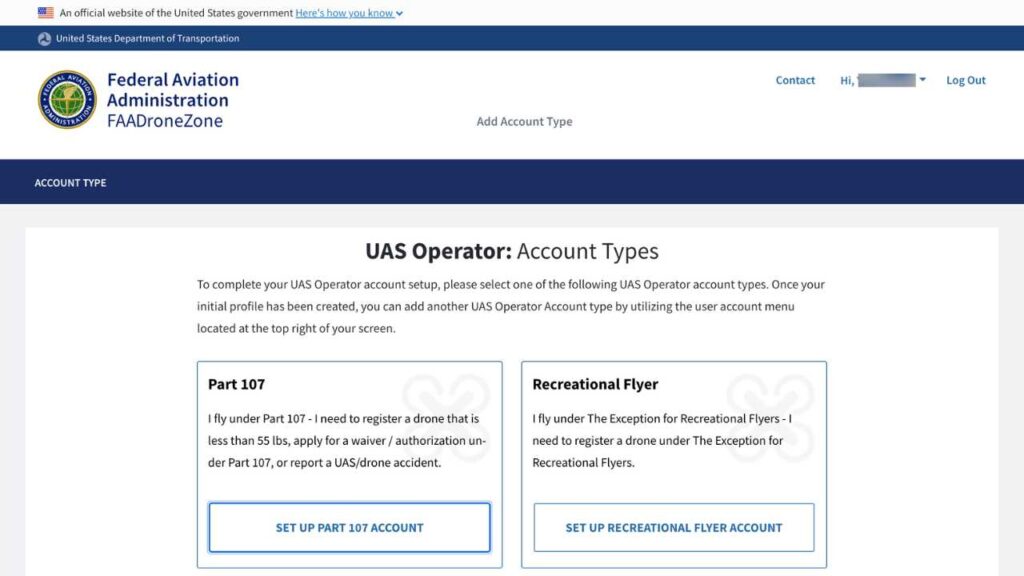This rectangular image is a screenshot of an official U.S. government website. In the upper left corner, there's a small American flag icon followed by the text "An official website of the United States government. Here's how you know," accompanied by a pull-down link for more information. Directly below, a black bar spans the width of the page and displays the text "United States Department of Transportation."

Underneath the black bar, a white banner features the logo for the Federal Aviation Administration (FAA), followed by the words "FAA DRONEZONE" prominently displayed. In the upper right corner of the image, options for "Contact" and "Logout" are visible, along with an "Add Account" button. Below this section, a blue bar runs horizontally across the page, housing the text "Account Type."

The main content appears on a white background. At the top, bold black text reads "UAS operator." Below this heading, two account type options are listed: "Part 107" and "Recreational Flyer." These options evidently correspond to different categories of drone operators.